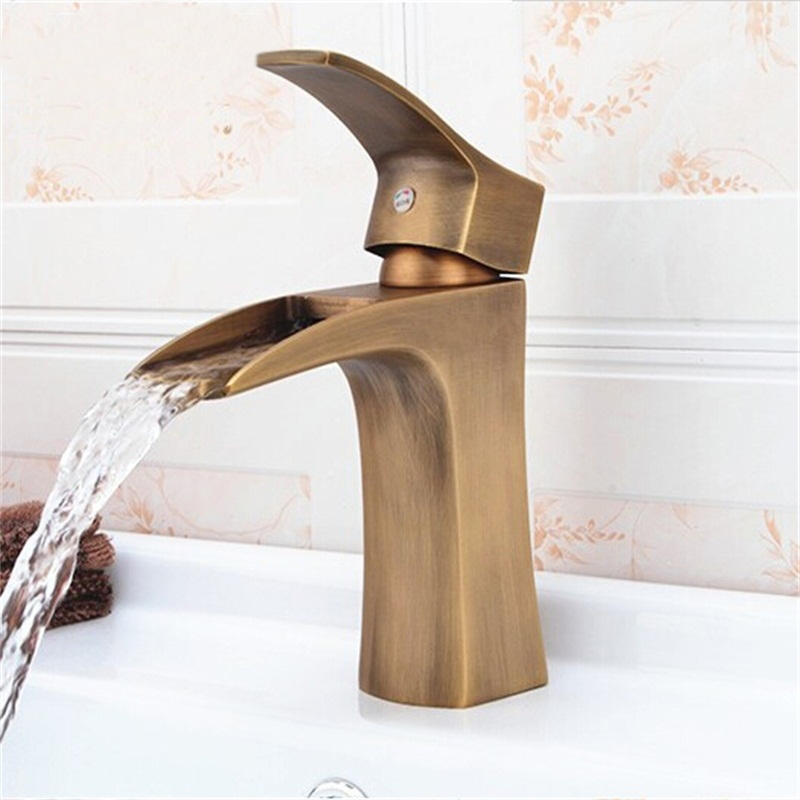This detailed photograph showcases a modern, brass-colored faucet with a unique design, situated in a bathroom setting. Water is seen pouring out from a horizontal slit, rather than a traditional spout, and is flowing into a white porcelain sink. The faucet features a lift handle on top to regulate the water flow, and the temperature appears to be set to a medium level, neither hot nor cold. In the background, there's a wall adorned with white tiles that have a delicate floral pattern in pink. To the left of the faucet, partially obscured by the steady stream of water, are brown towels. Additionally, small sponges can be noticed on the sink, likely intended for handwashing purposes. The overall aesthetic of the faucet and the sink suggests a modern, yet classic design element within the bathroom.